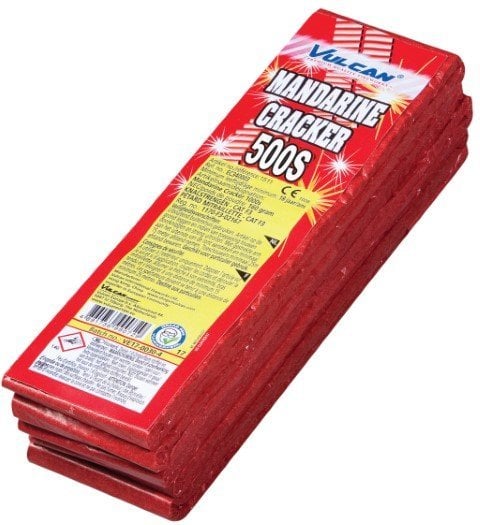The image depicts a red package of Vulcan Mandarin Crackers 500-S. The package is designed with a prominent "VULCAN" label in blue at the top, followed by "MANDARINE" in bold white capital letters outlined in black, and "CRACKER" beneath it. Further below, it states "500-S" and features a yellow rectangle with unreadable text, likely containing warnings or safety instructions. The bottom of the package displays a UPC barcode and additional warnings, along with a CE mark in the upper right corner, indicating compliance with safety standards. The package is red and rectangular, resembling the shape of a graham cracker. The image also shows five such identical red packages stacked on top of one another, all with similar labeling, characteristic of consumer fireworks from Vulcan Corporation.